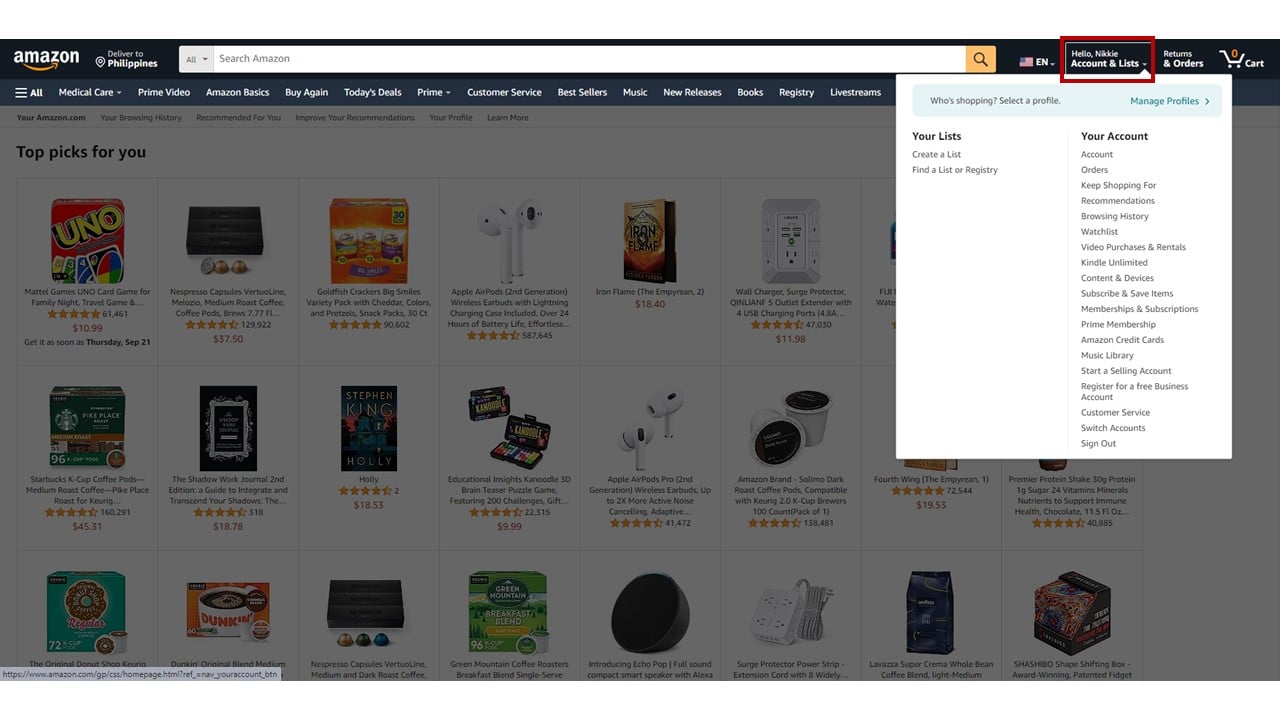This is a detailed screenshot of an Amazon.com webpage, featuring a prominently styled black banner at the top. On the far left of this banner, the Amazon logo is displayed in white alongside its signature gold smile. Positioned next to the logo, the text "Delivered to the Philippines" is visible. 

In the center, a broad search bar, labeled "Search Amazon," is situated for easy product searches. Adjacent to the search bar on the right, there is a magnifying glass icon, followed by an American flag with the letters "EN" indicating the site language is set to English. 

Further right, there's a red box enclosing the text "Hello, Nikki: Account & Lists," making it easily noticeable. To its immediate right are links for "Returns & Orders" and a shopping cart icon showing zero items.

Underneath the "Hello, Nikki: Account & Lists" section, a drop-down menu appears with options like "Who’s Shopping?" allowing users to select and manage profiles. 

On the left side of this drop-down, options include "Your Lists," "Create a List," and "Find a List or Registry." On the right side, more comprehensive account options are listed, including "Your Account," "Account," "Orders," and "Keep Shopping for." Additional sections cover "Recommendations," "Browsing History," "Watch List," "Video Purchases and Rentals," "Kindle Unlimited," "Content and Devices," "Subscribe & Save Items," "Memberships and Subscriptions," "Prime Membership," "Amazon Credit Cards," "Music Library," "Start a Selling Account," "Register for a Free Business Account," "Customer Service," "Switch Accounts," and "Sign Out."

In the background, a grayed-out section displays "Top Picks for You," showcasing a variety of recommended items for potential purchase.